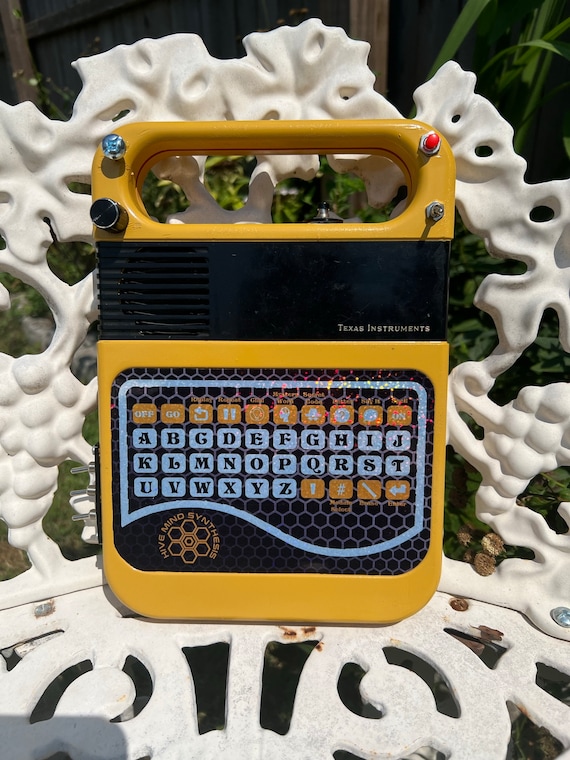This is a vertically aligned photograph featuring a yellow electronic device branded by Texas Instruments. Dominating the composition, the device includes a screen and an array of flat push buttons. These buttons are white squares with black letters arranged alphabetically from A to Z. Above the alphabetical keys, there is a row of orange function buttons labeled 'off,' 'go,' an arrow, and 'pause.' Notably, the device features a red button in the upper right corner and a blue-hued screw at the top. The top section also showcases a black horizontal frame with speaker ports and the Texas Instruments logo in fine print, beneath a yellow handle. The edges of the device are bordered in the same yellow material, which appears to be a mix of plastic and metal. The whole setup rests on what seems to be a white, ornate, wrought iron surface, possibly a bench or chair, against a backdrop that includes a wooden fence and some plants, adding an outdoor ambiance to the shot.